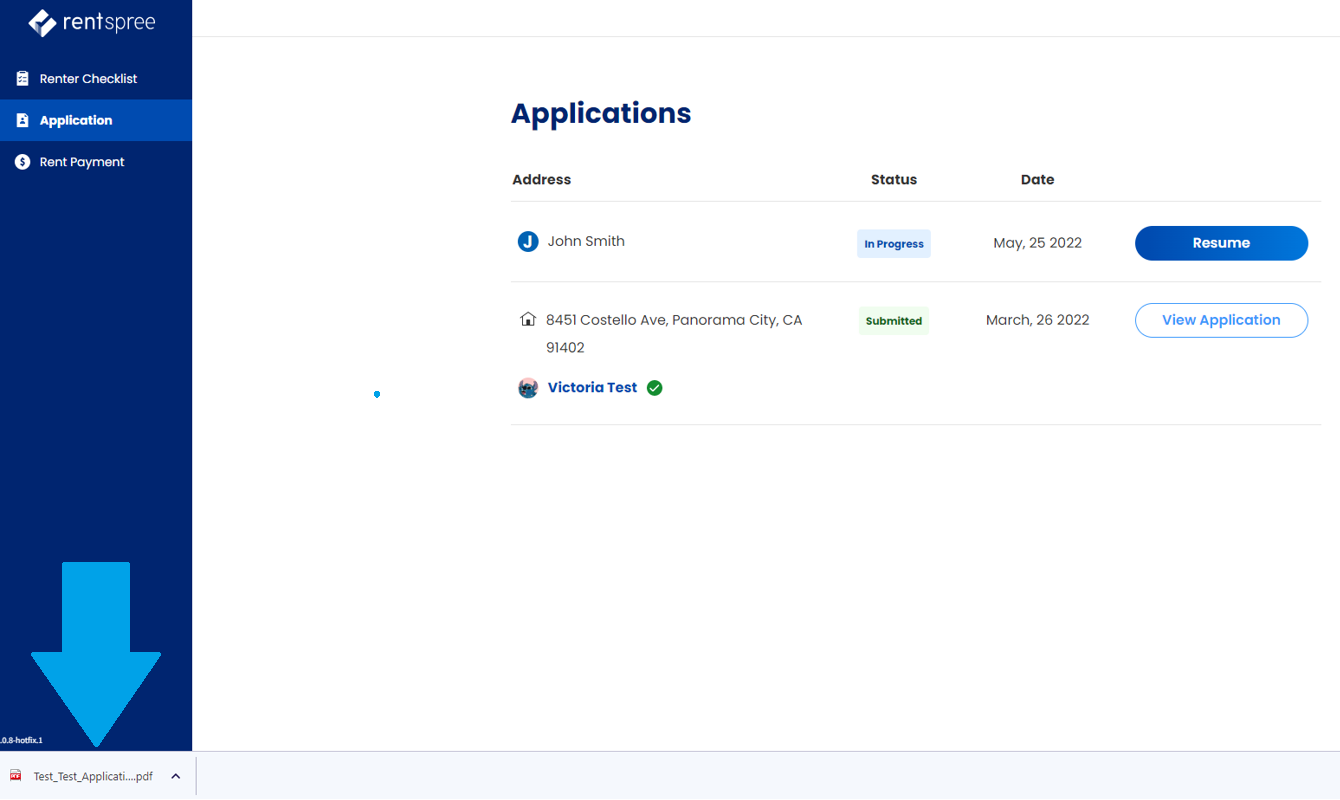In this image, the interface of a web application is divided visually into two distinct sections. The left side, occupying one quarter of the page, features a dark blue background with the "Rent Spree" logo prominently displayed in white at the top left corner. Below the logo are three sections: "Renter Checklist," "Application," highlighted with a lighter blue background and white text, and "Rent Payment." At the bottom of this sidebar, a light blue arrow points downwards, suggesting additional options or information.

The remaining three quarters of the page have a clean white background. At the top, the dark blue heading "Applications" stands out. Directly beneath this heading are columns labeled "Address," "Status," and "Date." 

The content is organized as follows:

1. **First Line:**
   - **Address:** Featuring the name "John Smith" displayed next to a blue circle with a white "J" in the center.
   - **Address Details:** "8451 Costello Avenue, Panorama City, California, 91402."
   - **Status:** A homeowner verification with a house icon followed by the text "Victoria Test" in blue, accompanied by a green check mark.
   - **Application Status:** "In Progress."
   - **Submission Status:** "Submitted."
   - **Dates:** "May 25, 2022" and "March 26, 2022."
   - To the far right, there is a prominent blue button labeled "Resume."

2. **Second Line:**
   - A white button labeled "View Application" is positioned underneath the first line’s blue button.

The detailed layout and color scheme guide the user's interaction with the webpage, making navigation and application status tracking intuitive and visually distinct.